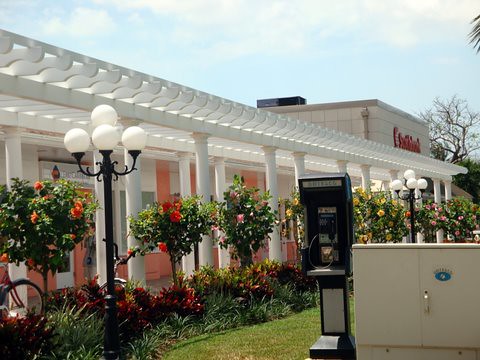The photo captures an outdoor walkway beneath a white pergola with smooth Doric columns against a salmon-colored stucco wall, part of a strip mall reminiscent of Florida's typically lush, overlandscaped aesthetic. Hibiscus plants line the walkway, showcasing a variety of vibrant colors. Towards the right, beneath the pergola, stands a black payphone—a rare sight nowadays—in front of a metallic gray utility box with a silver handle. A stylized lamppost with four white globes is situated to the left, adding to the ornate decor. The background features the upper facade of a large building, possibly a store, adorned with a red-lettered logo that's partially obscured.